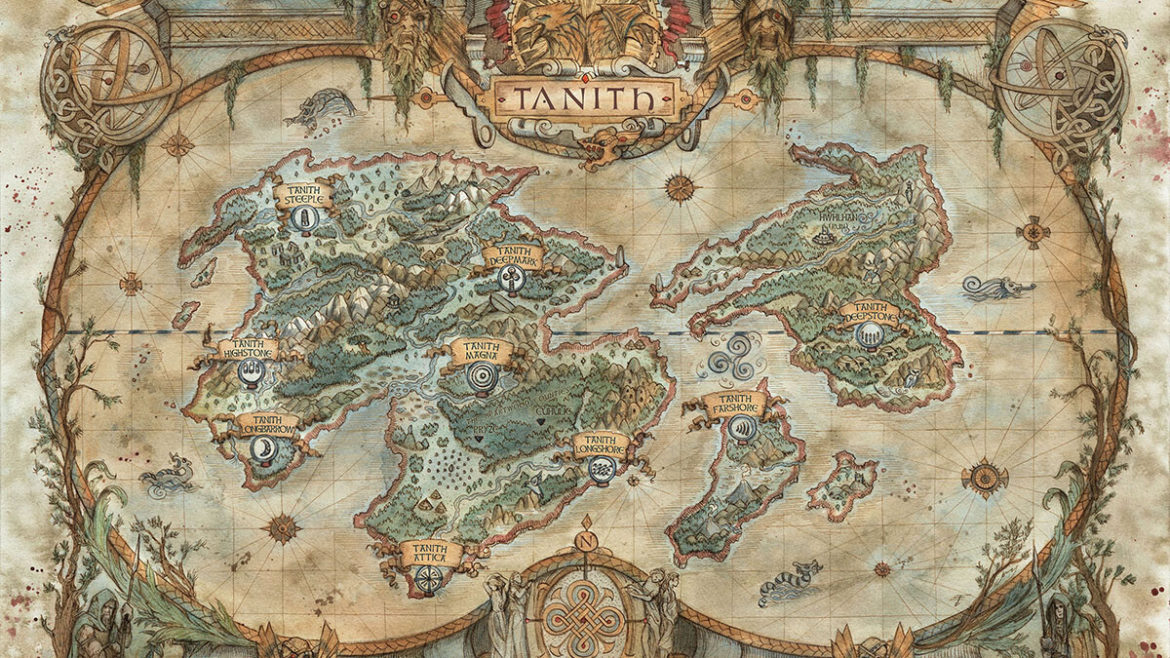This illustration depicts an archaic, discolored map labeled "Tanith" at the top in prominent, non-English letters. The map, reminiscent of Greek mythology and old-world designs, is filled with intricate, descriptive illustrations of lands scattered across a singular lurid area. The layout of the map forms almost a figure-eight or two intertwining circles, with islands dotting the water, which features fish and a notably windy area depicted by swirling designs. Faces adorned with jewel-like eyes add a statue-like quality to the artwork. Vines and ivy creep along the edges, enhancing the ancient feel. Various locations are labeled, though the names are mostly undecipherable except for “Tanith Steeple.” The map's rich colors—dark green, goldish yellow, and aged beige—contrast with its aged appearance, making it look like something you'd find in a fantasy novel, guiding readers through a fictional world.